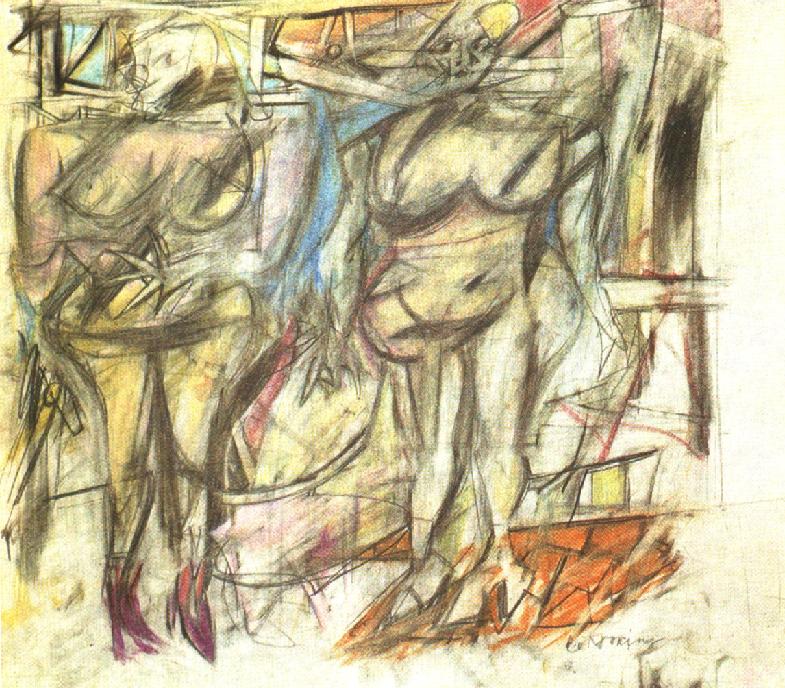This is a detailed colored pencil sketch with elements of futuristic art and modern cubism, featuring a complex cityscape backdrop. Predominantly in cobalt steel blue with accents of red, yellow, orange, and geometric patterns, this large square drawing has no defined border. The primary subjects are two female figures centrally positioned among a flurry of black charcoal scribbles and slashes. 

The figure on the left appears nude with large breasts, a smiling, alien-like face, and possibly blonde hair indicated by yellow markings near the head. The right-side figure also appears nude with larger breasts, a visible belly button, legs, and bare feet positioned on a geometric orange ground. The chaotic background includes indistinct body parts and faces, making it challenging to differentiate specific details amidst the abstract forms. 

Towards the top, there's a yellow light bulb, contributing to the enigmatic ambiance. The lower right corner features the artist’s signature, though it remains difficult to decipher. The overall texture of the piece affirms extensive use of colored pencils complemented by smudged charcoal, resulting in a visually intricate blend of humanoid forms and abstract shapes.